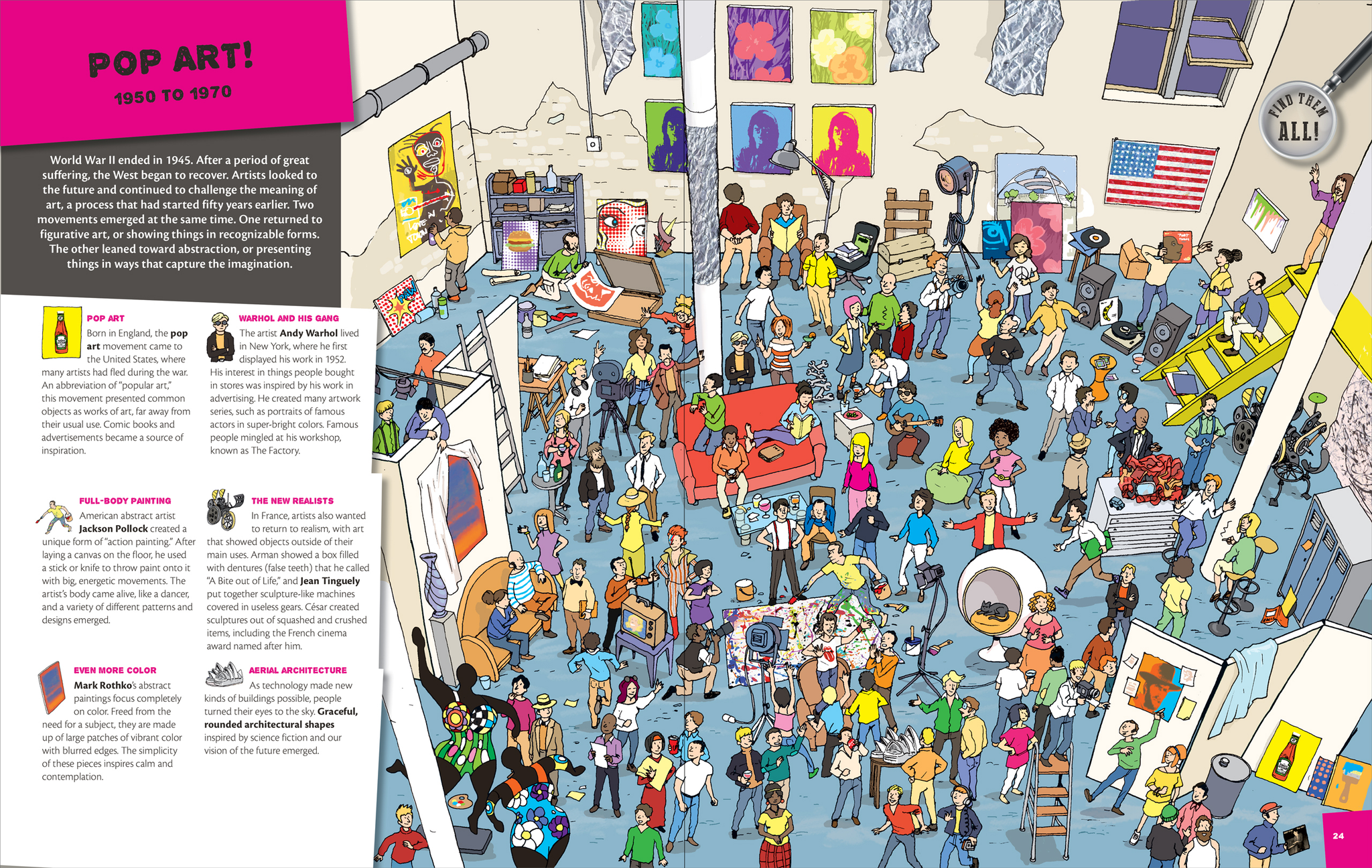This image appears to be from a magazine article titled "Pop Art, 1950-1970" and features a blend of text and a colorful, cartoonish drawing. The left side of the image contains sections of text laid out on a pink and gray background. The pink section at the top states the title "Pop Art, 1950-1970," and below it, a gray box details the post-World War II art movements, describing how artists challenged the meaning of art, splitting into two main movements: figurative art and abstraction.

The detailed paragraphs on the left cover different themes and artists of the Pop Art era. One titled "Pop Art" explains the movement's origins in England and its transition to the United States, showcasing common objects as art. Another paragraph on "Full Body Painting" highlights Jackson Pollock's energetic abstract painting techniques. "Even More Color" describes Mark Rothko's focus on large patches of vibrant color, and "Warhol and his gang" recounts Andy Warhol's influence in New York, his fascination with consumer goods, and his famous workshop, The Factory. "The New Realist" discusses French artists' attempts to return to realism with quirky, everyday objects, and "Aerial Architecture" touches on futuristic, rounded architectural designs inspired by advances in technology.

On the right side, the image showcases a brightly colored, cartoon-like drawing depicting an art museum scene. The room has beige walls and a blue floor, filled with hundreds of people engaged in various activities. Some are painting, taking photos, playing guitars, reading books, dancing, or simply talking. The diverse group of people wearing different colored clothes adds to the dynamic and vibrant atmosphere, capturing the essence of the Pop Art era and its impact on society and culture.